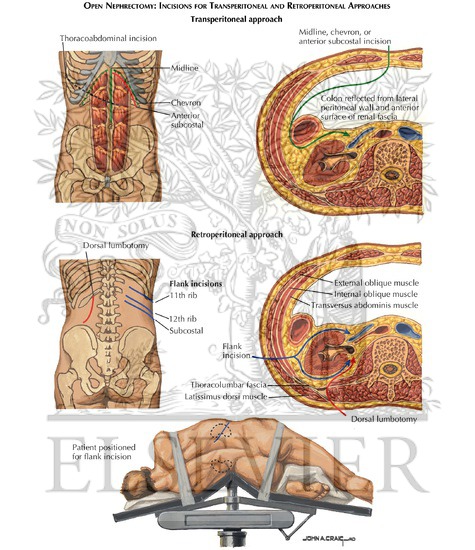The poster illustrates various surgical techniques and patient positioning methods for nephrectomy, specifically through transperitoneal and retroperitoneal approaches. The background is white with prominent black text at the top reading, "Open Nephrectomy Incisions for Transperitoneal and Retroperitoneal Approaches."

The upper section is divided into two main areas:

1. **Transperitoneal Approach**:
   - On the left, a detailed illustration shows a thoracoabdominal incision marked on a torso. Labels point to various anatomical landmarks like the "midline" and the "anterior subcostal."
   - To the right, a closer view highlights the incision methods, marked by green lines pointing to terms such as "Midline Chevron" and "Anterior Subcostal Incision."

2. **Retroperitoneal Approach**:
   - On the left, another detailed illustration shows an incision line extending from the top of the hip bone upwards, labeled "dorsal lobotomy." Additional labels point to anatomical structures like the "11th rib," "12th rib," and "subcostal."
   - To the right, a detailed cross-sectional view highlights the incision area with a blue line circling around the "external oblique muscle," labeled as a "flank incision."

At the bottom of the poster, there's an image demonstrating the patient positioning for a flank incision. The patient is shown naked and lying on their side, strapped to a specialized table. The table has a gray, triangular support that raises the torso, making the spine arch and creating better access for surgeons.

The detailed color illustrations use flesh tones for the skin, lighter shades for bones, and orange hues for organs, providing a clear visualization of the surgical procedures and anatomical structures involved. This comprehensive poster offers a clear educational overview of the specific surgical approaches and positioning techniques used in nephrectomy.